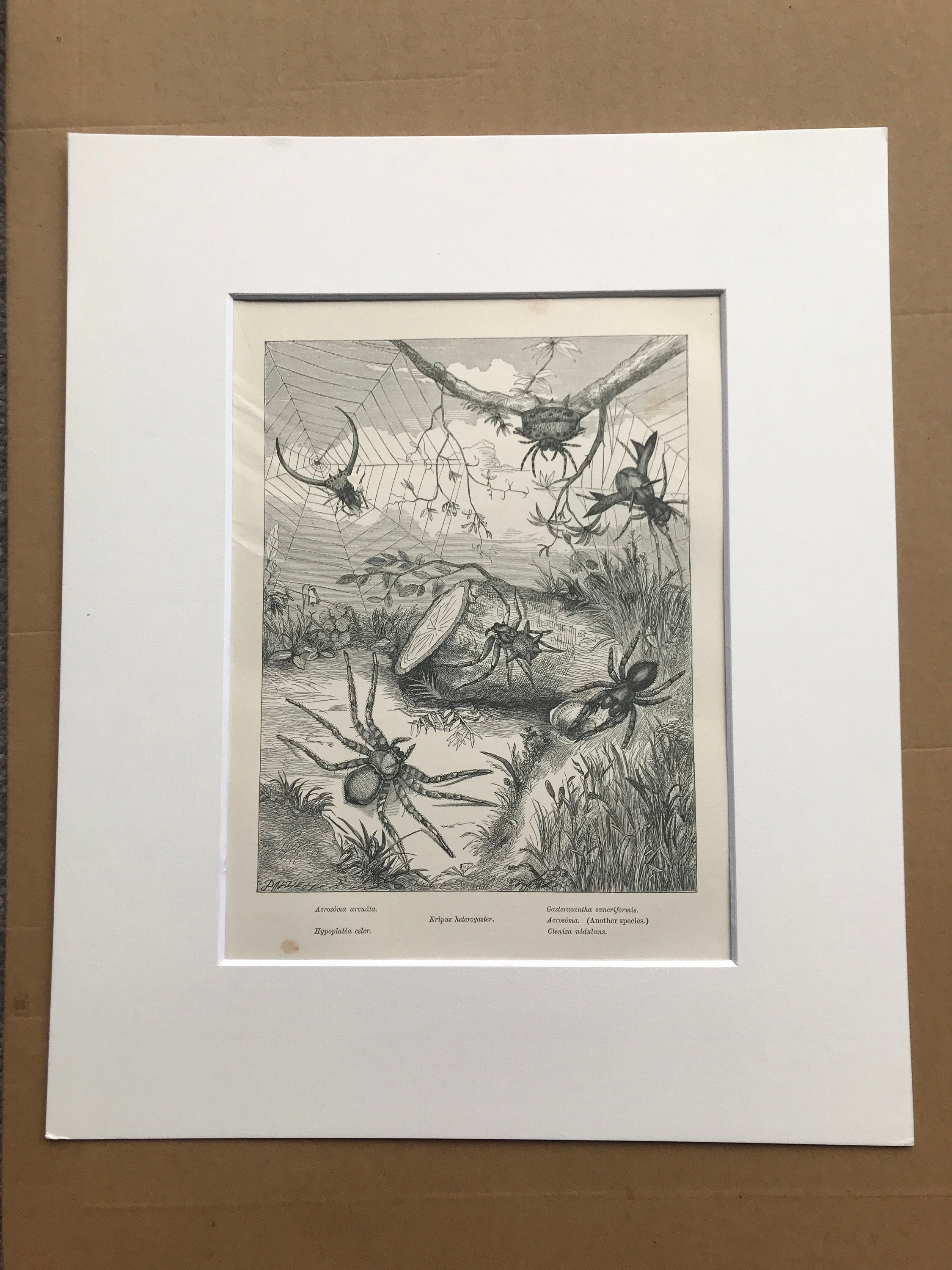This image appears to be a close-up photograph of a framed black-and-white drawing featuring six large spiders, possibly tarantulas, along with smaller spiders. The detailed illustration also includes spider webs, a hanging branch, grass in the foreground, a log, and a patch of dirt in the middle of the composition. This intricate drawing is contained within a tall, raised white rectangular border that is itself set against a brown background, perhaps suggesting it is on display in a museum. There are descriptions below the graphic, though they are too small to read. Overall, the artwork and its unique presentation stand out clearly.